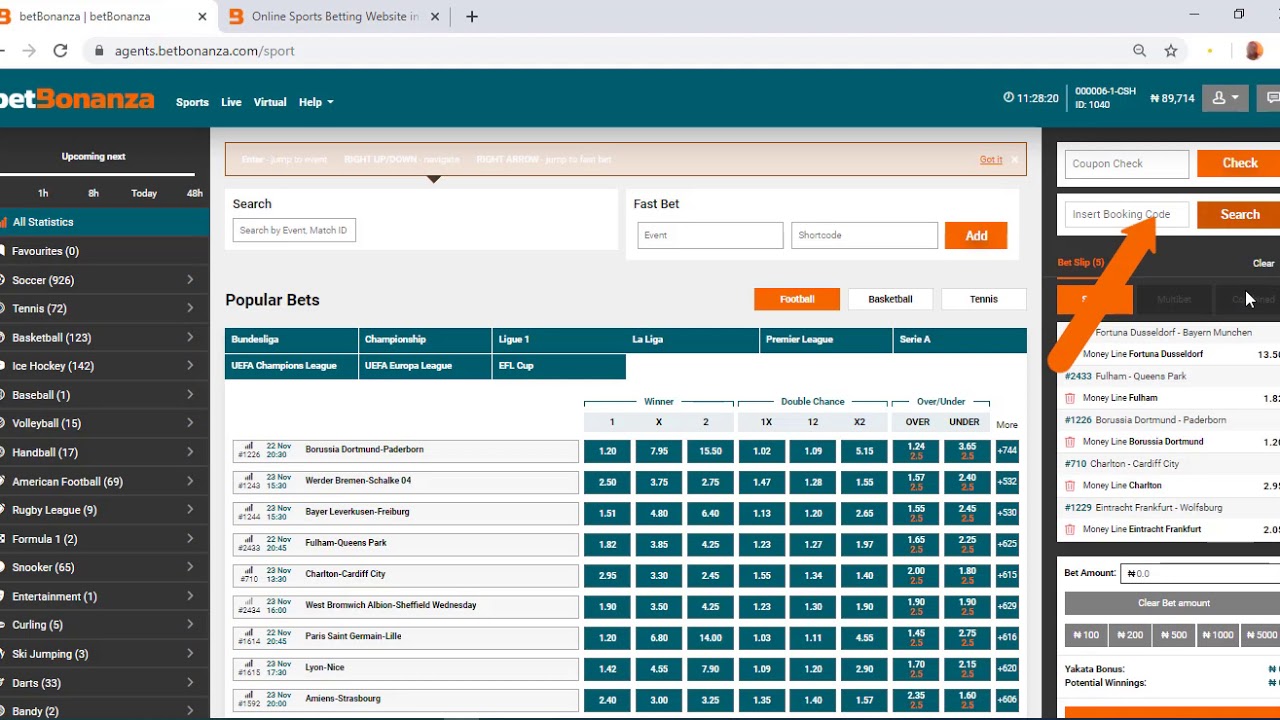A screenshot of the BetBonanza website highlights its user interface and various features. The browser displays two tabs: "BetBonanza" and another tab partially truncated as "Online Sports Betting Website". The address bar shows the URL: agents.betbonanza.com/sport.

At the top of the site, the BetBonanza logo is prominently featured with "Bet" in white and "Bonanza" in orange. The menu bar to the right includes buttons labeled "Sports", "Live", "Virtual", and "Help" with a dropdown arrow. A clock on the menu bar shows the time as 11:28:20, presumably in hours, minutes, and seconds. There is also a partially blurred ID, an "N" with a horizontal line and the number 89,714 next to it. Additionally, there is a square button featuring a silhouette of a person with a dropdown arrow and another button resembling a comment symbol, commonly seen in cartoons, albeit very small.

The screen is divided into three columns. The left column is labeled "Upcoming" and "Next" and includes various sports categories, alongside filtering options like "Hour", "8 Hours", "Today", and "48 Hours". The central column allows users to search by event, match ID, fast bet, or event short code. Popular bets are categorized under football, basketball, and tennis. The rightmost column features a "Coupon Check" section with an option to insert a booking code for further actions.